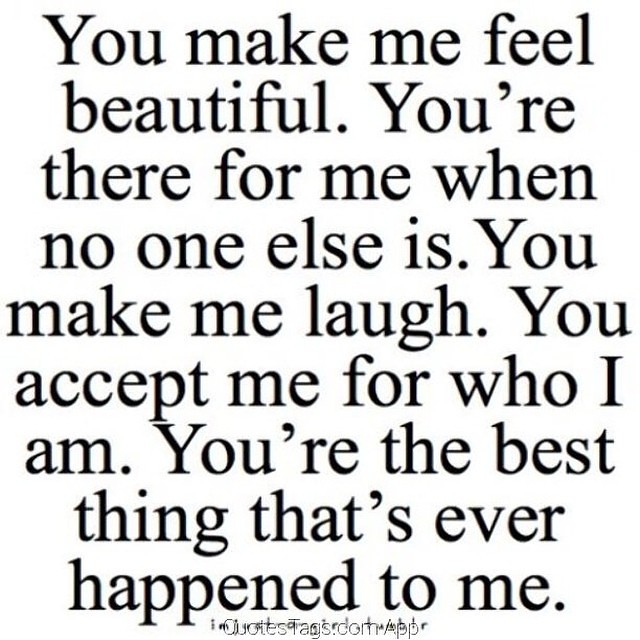The image features a heartfelt quote from Quotetags.com/app, saying, "You make me feel beautiful. You're there for me when no one else is. You make me laugh. You accept me for who I am. You're the best thing that ever happened to me." This emotionally charged message speaks to the deep love and appreciation someone feels for another, highlighting themes of support, laughter, acceptance, and gratitude. The presentation of the quote suggests it could be used on various platforms like t-shirts or social media sites such as Facebook or Instagram. However, there appears to be a slight design issue with the text, where attribution details from the website overlap with the quote itself, making it a bit difficult to distinguish the source.